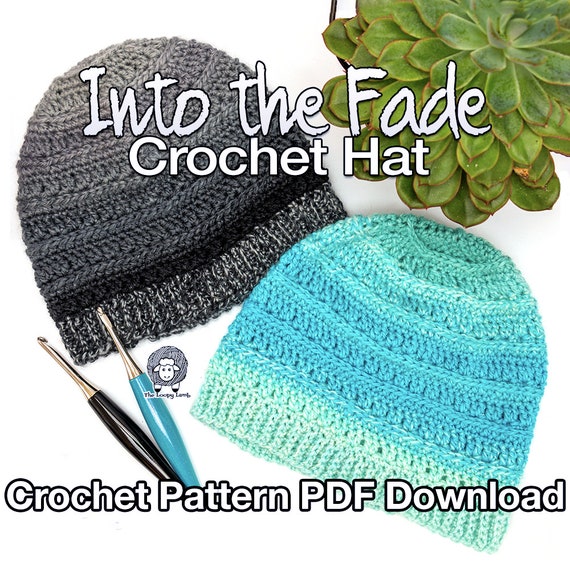The image appears to be a promotional advertisement for a knitting business, prominently featuring two beanie-style crocheted hats with gradient color schemes. The hat on the left transitions from black to light gray, while the one on the right shifts from light blue to a teal greenish-blue. At the top of the image, white text reads "Into the Fade Crochet Hat," with "Crochet Pattern PDF Download" at the bottom. To the right, a small succulent with tiny green leaves adds a touch of greenery. The logo, a cartoon sheep with the text "The Loopy Lamb," is displayed, likely representing the business. Also shown are two crochet tools, indicating their use in creating these patterns.